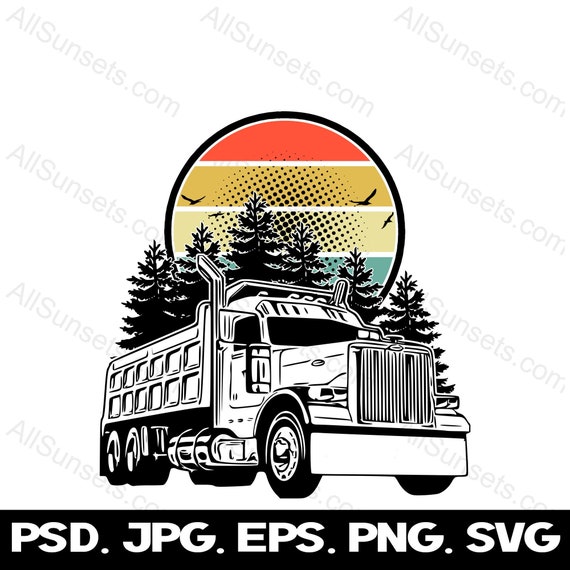This digital art piece from allsunsets.com showcases a semi-truck set against a vivid, multi-layered sunset backdrop filled with hues of orange, yellow, beige, green, and blue. The scene is enclosed within a circle that features dotted patterns adding depth to the design. Silhouetted evergreen trees create a picturesque foreground, giving the impression of a truck hauling Christmas trees. Above the truck, birds are seen soaring, further enriching the composition. The bottom of the image bears a black sign listing various file formats available for download—PSD, JPEG, EPS, PNG, SVG—indicating its versatility for use as labels, tattoos, or other creative applications. The watermark across the piece ensures visibility of its source, allsunsets.com, emphasizing its online availability.